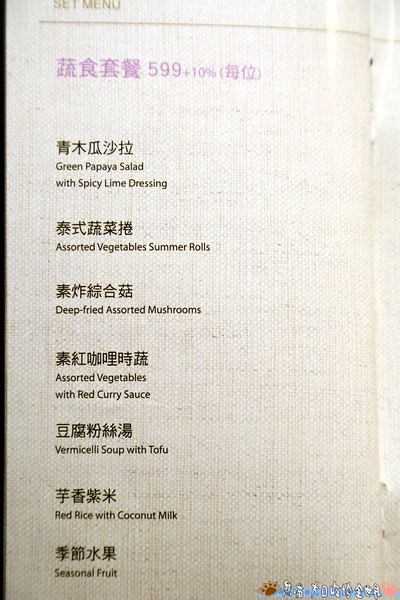The image displays an elegantly designed menu on a white, textured linen-like background. At the top, the words "Set Menu" are inscribed in a faded pink hue, followed by a thin yellow line stretching across the width of the menu. Below, the menu items are listed, each title written in bold oriental script, likely Chinese or Japanese. Each item is paired with an English description beneath it. The items include: green papaya salad with spicy lime dressing, assorted vegetable summer rolls, deep-fried assorted mushrooms, assorted vegetables with red curry sauce, vermicelli soup with tofu, red rice with coconut milk, and seasonal fruit. Notably, "599 plus 10%" is also indicated alongside the text. The left edge of the menu features a distinctive black border, giving the menu a sophisticated and organized appearance.